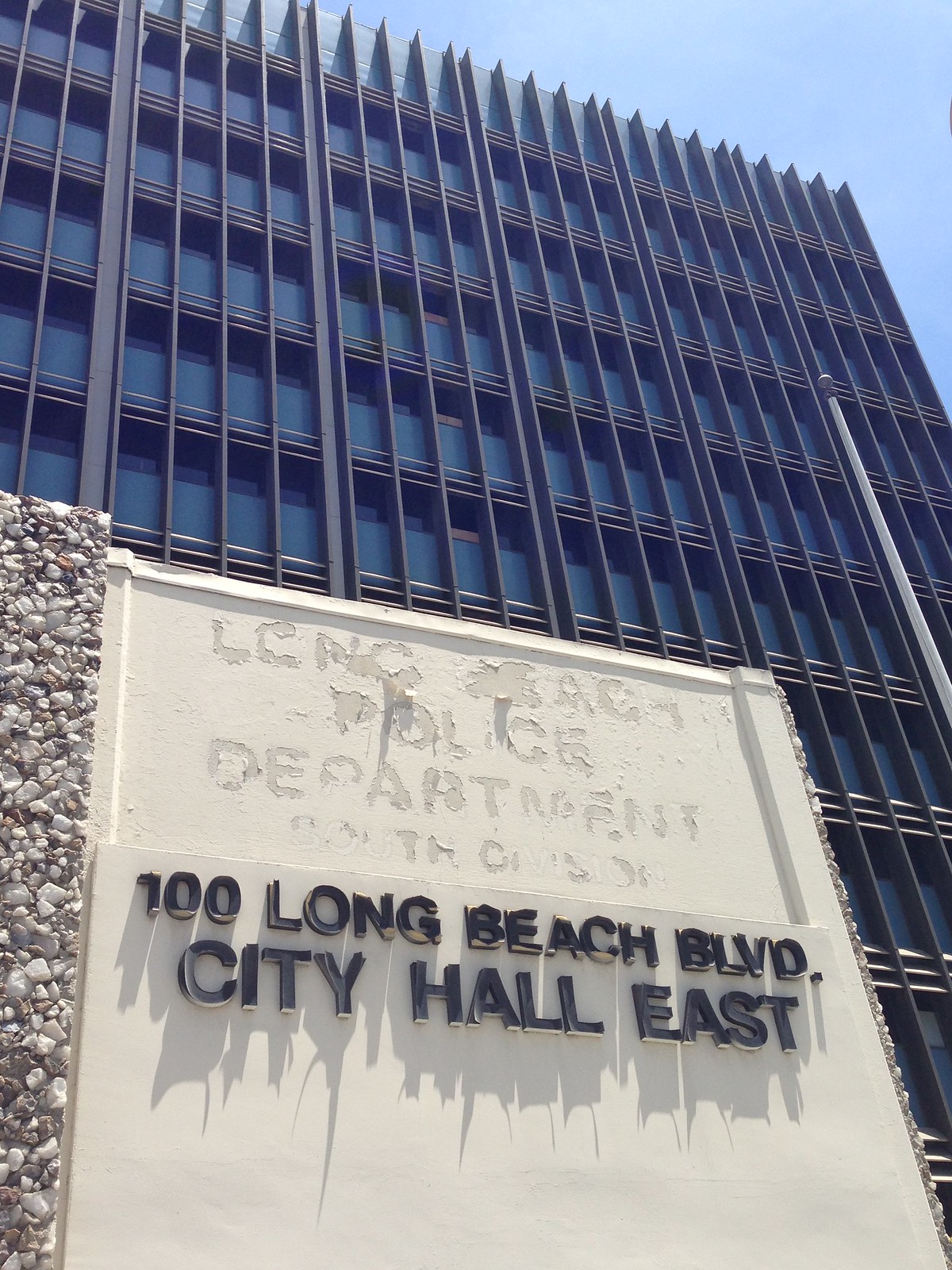The image, taken from street level on a sunny day, captures a large office building that rises at least seven to nine stories high, though it could be as tall as six stories. The facade is marked by numerous windows separated by tall steel beams. A flagpole without a flag is visible on the right-hand side of the photograph. Dominating the foreground is a large cement sign, flanked by rocky pillars, which clearly displays the address "100 Long Beach Boulevard, City Hall East" in three-dimensional black letters. Above this address, the remnants of an older sign read "Long Beach Police Department South Division," though the lettering is weathered and partially faded. To the left of the sign, you can see a wall made of stones and cement. The sun casts its light warmly over the scene, emphasizing the details of the building and the surroundings.